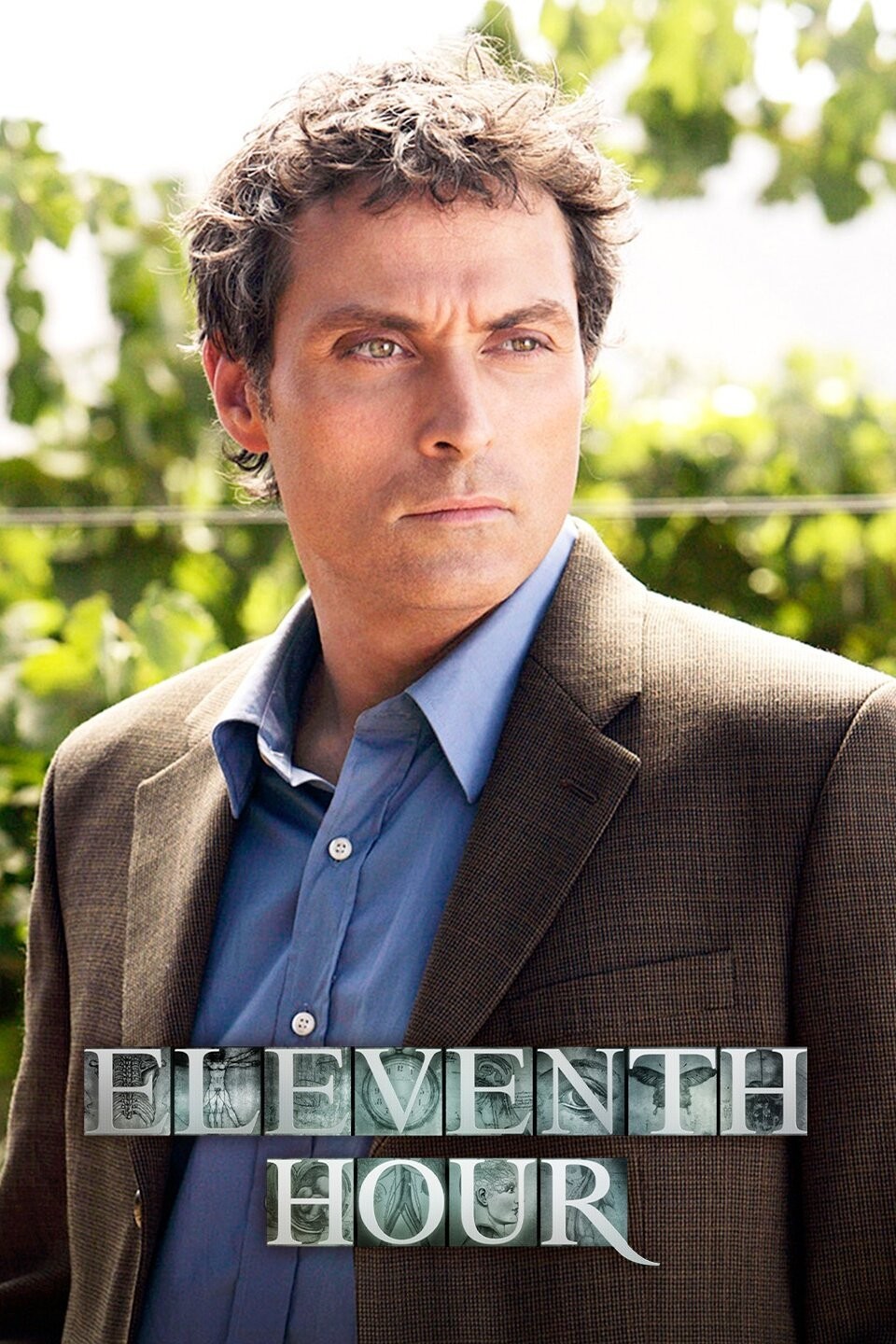The image appears to be a promotional photograph, possibly for a movie or a show, showcasing a man with short, curly brown hair that seems to have gray or white highlights. He has thick eyebrows and light brown eyes, with a clean-shaven face. The man is dressed in a blue dress shirt, which is buttoned up except for the top button, and a brown tweed blazer. He stands facing somewhat towards the left side of the image, looking sternly into the distance as if pondering something.

The background features blurred vegetation with green leaves and trees, indicating an outdoor setting on a bright, sunny day, with sunlight illuminating some objects in the picture. Additionally, the background includes some white lights, possibly from the sun or other light sources.

Prominently displayed at the bottom part of the image is the text "11th hour" in bold, white capital letters. Each letter is within individual rectangular or square blocks with a greenish-blue background that contains various symbols: one has an eyeball, another might show a clock, and another depicts the spread wings of an insect or bird. The man’s stern expression and the specific details in the background suggest a high-quality promotional image intended to captivate potential viewers.